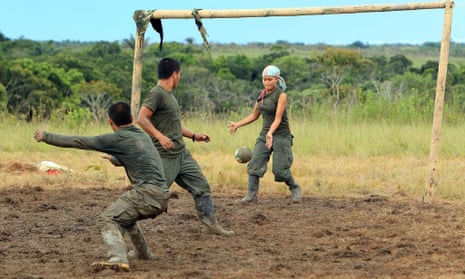In this photograph, three individuals dressed in dark olive green military-style attire are engaged in a game of soccer on a muddy, makeshift field set in a wilderness area. On the left, a man sports a dark olive green long-sleeved shirt, while the man in the middle is clad in a short-sleeved crewneck shirt of the same color. Both are covered in mud, indicative of vigorous activity. To the right, a woman stands as the goalkeeper, centered within a goal constructed from three long branches forming a rectangular shape. She is outfitted in a sleeveless olive green t-shirt with cargo pants, and she wears a light blue bandana on her head paired with a red scarf around her neck. The woman’s boots match the military fatigues of the men, who are also wearing similar dark olive green cargo pants tucked into their boots. She appears ready to catch or kick a ball that is mid-air in front of her, with her arms outstretched and legs poised. The scene captures a moment of intensity and teamwork amidst a rugged, natural backdrop.